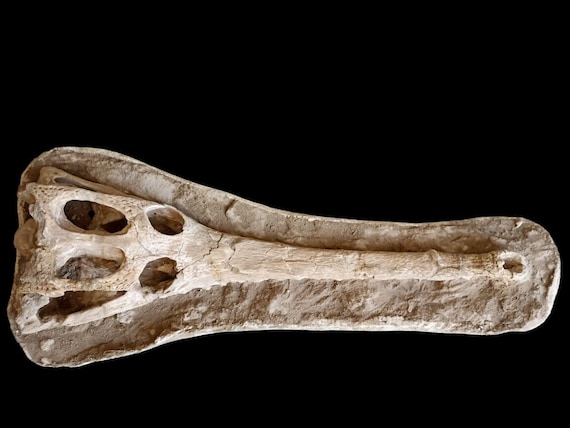The image depicts a bone against a black background. The bone has a slightly darker whitish color on the exterior and exposes its inner structure in some areas. The left side of the bone is wider and features five distinct holes: three elongated, horizontal ones aligned parallel, and two more circular holes positioned diagonally above and below, slightly angled towards the left. The bone tapers towards the right, ending in a curved shape reminiscent of a paw, possibly from a cat or dog. Near the bottom of this paw-like structure is another small hole, suggesting a point where another part of the bone or tissue might have once been attached. The overall texture shows visible cracks, accentuating its aged and worn appearance. The bone's unique shape could be interpreted as either resembling a primitive tool with a handle or part of an animal's foot, though it's predominantly speculated to be just an old bone.